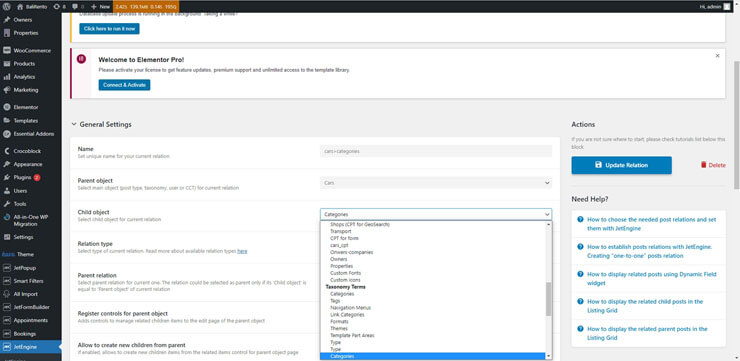This image depicts the settings section of a WordPress website. The interface showcases a black left sidebar containing multiple tabs, numbered sequentially from 1 to 24. The 24th tab is highlighted, but the specific label is unreadable. At the top, there is a home tab situated in the top border of the screen.

To the immediate right of the sidebar, the main settings panel is visible. Within this panel, there are various buttons; one notable button includes the partial text "Welcome to X Eliminator Prop,” adjacent to which is a button marked by a red circle enclosing a closeout square. 

The primary section of the page is dominated by general settings. This area includes textual fields or settings such as "Prevent Object" and "Child Object," and three additional unreadable labels. There is a dropdown box that appears to provide multiple language options, currently set to the first choice, though the exact language is not discernible.

Additionally, there is a feature related to updates signified by an "Update Resolution" or "Update Request" box positioned next to a red trash can icon.

At the bottom of the settings panel, there is a "Need Help" section listing five entries, presumably providing support or FAQ topics.

This detailed layout ensures easy navigation and accessibility on the settings page of the WordPress site.